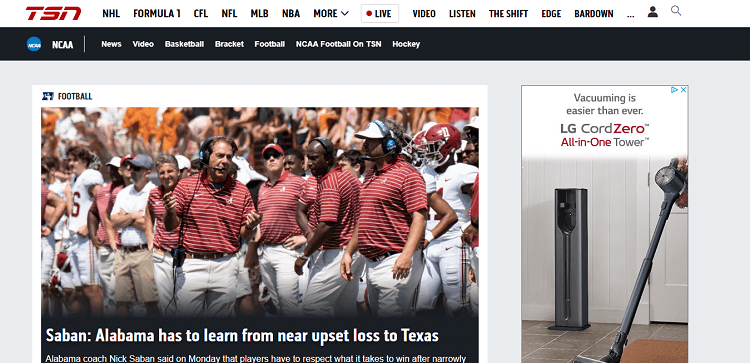The TSN website homepage prominently displays a variety of sports categories including NHL, Formula One, CFL, NFL, MLB, NBA, and more. The navigation bar, arranged from left to right, includes sections such as Live, Video, Listings, The Shift, The Edge, and BarDown. Underneath this main navigation, there is a black banner box featuring the NCAA logo followed by links for News, Video, Basketball, Bracket, Football, NCAA, Football on TSN, and Hockey.

Below the banner, a prominent photograph captures an American football scene. The image shows fans and players in the background, along with six coaches who are dressed in red and white striped polo shirts and white pants. At the bottom of the image, a headline reads, "Saban: Alabama has to learn from near upset loss to Texas. Alabama coach Nick Saban said on Monday that players have to respect what it takes to win after narrowly..." The sentence remains incomplete.

To the right of the photo, an advertisement for LG is visible, showcasing the LG CordZero All-In-One Tower vacuum cleaner. The ad highlights the convenience of vacuuming with this tower-style vacuum cleaner, suggesting that LG is promoting the ease of use and efficiency of their product.